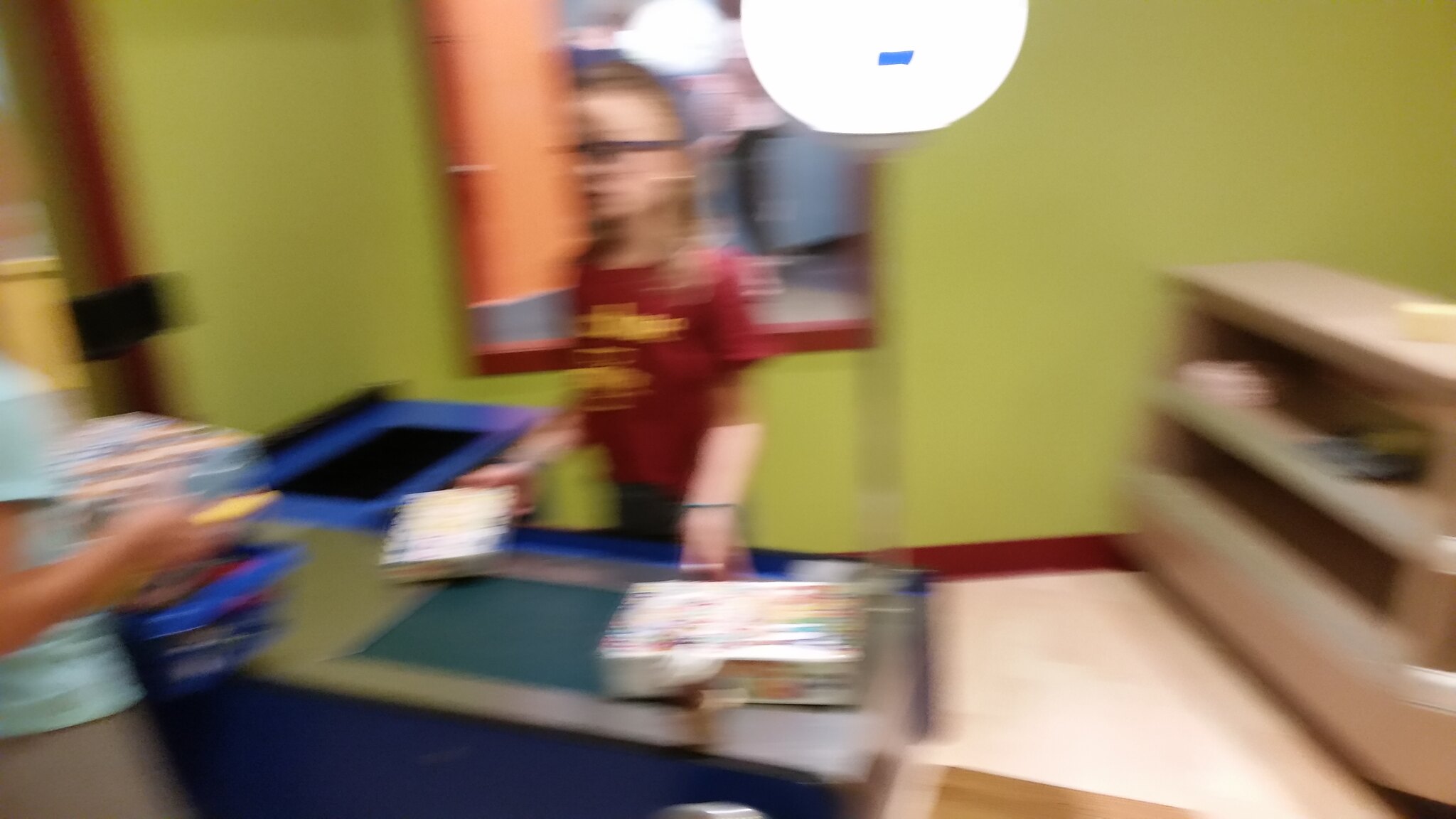In this slightly blurry image, the setting appears to be a school or classroom. A woman with blonde hair, wearing black glasses and a red shirt with yellow lettering, stands in front of a counter. She holds a book or box, possibly a game, in her right hand. To her right, there's a blue trash can with an open lid and a trash bag inside. On the left side of the image, another woman is partially visible; though her face is obscured. She holds a blue book along with a stack of other books in her left arm, and a yellow pen or marker in her right hand, suggesting she is engaged in a conversation with the first woman. The scene hints at an educational environment, perhaps during a preparatory or casual moment in the classroom.